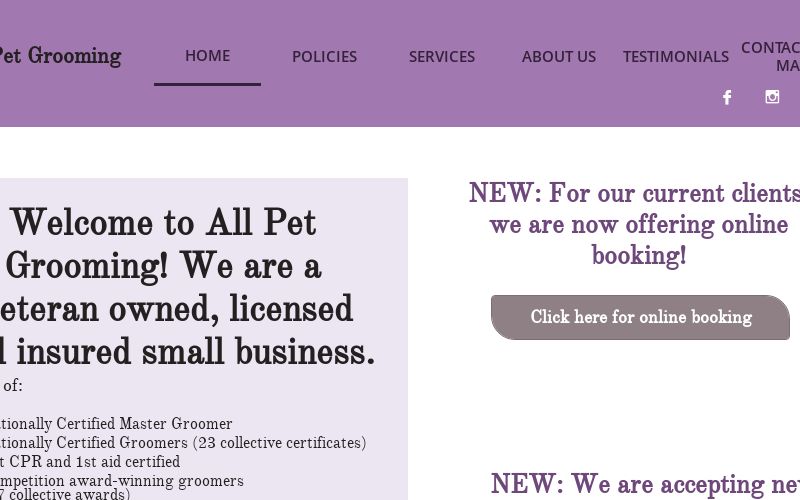The screenshot depicts a vibrant pet grooming website, predominantly featuring a clean white and purple color theme. At the top of the site is a bold purple banner laden with several navigational options including "Home" (which is highlighted), "Policies," "Services," "About Us," "Testimonials," and "Contact." Social media icons for Facebook and Instagram are situated alongside these menu items.

The main section of the webpage welcomes visitors with "Welcome to All Pet Grooming" in large, inviting text. It proudly boasts that the business is "veteran-owned, licensed, and insured," although part of the text is cut off. The snippet available highlights their credibility with phrases like "certified master groomer" and "23 collective certificates," hinting at their extensive expertise.

To the right, there is a noticeable call-to-action section for existing clients that announces, "We are now offering online booking." A button labeled "Click here for online booking" provides a direct link to this new service. It also hints at new offerings with a partially visible message starting with "New, we are accepting," though the remainder is obscured.

While no images of pets are present, the website heavily emphasizes textual information and links designed to navigate deeper into the site's content, ensuring visitors can easily access further details about their pet grooming services.